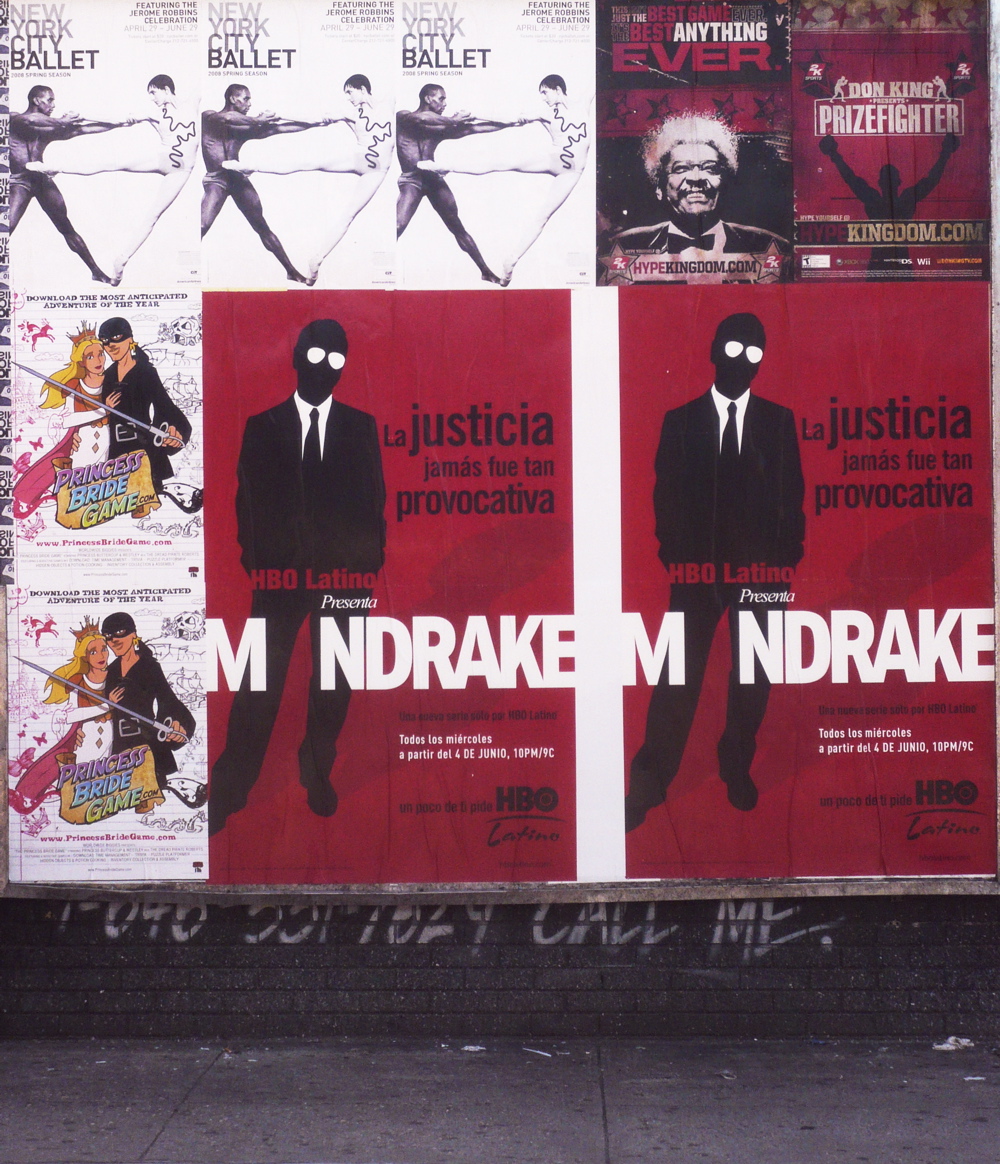In the photograph, a bustling street scene is centered around a brick wall adorned with an array of vibrant posters, situated beside a dark gray sidewalk. A blend of intriguing images and texts, the wall serves as a canvas for various advertisements and graffiti. Notably, the top left corner showcases three posters for the New York City Ballet, each depicting two dancers—one black and one white—against a white background. Below these ballet posters is graffiti with an unreadable phone number, suggesting "Call Me."

To the right of the ballet posters, a poster for Don King features prominently, promoting HypeKingdom.com with a bold, enthusiastic declaration about being the "best game ever." Adjacent to this is another Don King-related poster for "Prizefighter," blending a red and black color scheme, indicative of its intense boxing theme.

Lower on the left side, there are two posters for a Princess Bride-themed game, featuring cartoonish renditions of characters such as the Dread Pirate Roberts and the Princess, with a white backdrop. Dominating the right side of the wall are two striking posters for the HBO Latino-presented TV show "Mandrake," with vivid red backgrounds and styled akin to Mad Men art, titled "Mandrake: La Justicia, Jamara, Tu Provocativa."

Overall, the scene captures the juxtaposition of art and advertisement in an urban environment, reflecting both cultural events and popular media through a diverse palette of colors and styles.